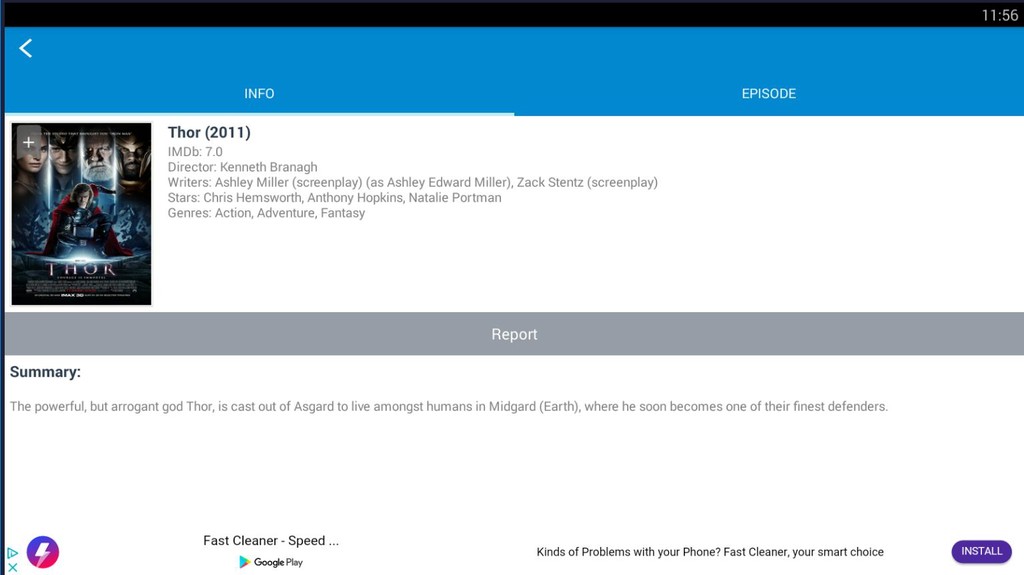This is a detailed screenshot of a website. At the top, there is a black bar with a timestamp reading 11:56 in the upper right corner. Below the black bar, there is a blue rectangle. In the upper left corner of this blue bar, there is a small white arrow pointing to the left. The blue bar features two tabs: "Info" and "Episode" in white font. The "Info" tab is selected, indicated by a small white line underneath it.

Below the blue bar, there is a white rectangle containing detailed information about the movie "Thor" from 2011. On the left side of this rectangle, there is the cover art of the movie "Thor," depicting the characters engaged in scenes typical of the film. Beneath the cover art, the word "Thor" is displayed.

To the right of the cover art, there is comprehensive information about the movie, including:
- Title: Thor (2011)
- IMDb rating: 7.0
- Director: Kenneth Branagh
- Writers: Ashley Miller (screenplay as Ashley Edward Miller) and Zack Stentz
- Stars: Chris Hemsworth, Anthony Hopkins, Natalie Portman
- Genre: Action, Adventure, Fantasy

Below this information, there is a gray bar with the word "Report" centered in white font. Beneath the gray bar, there is another section labeled "Summary" in black font on a white background. The summary reads: "The powerful but arrogant God Thor is cast out of Asgard."